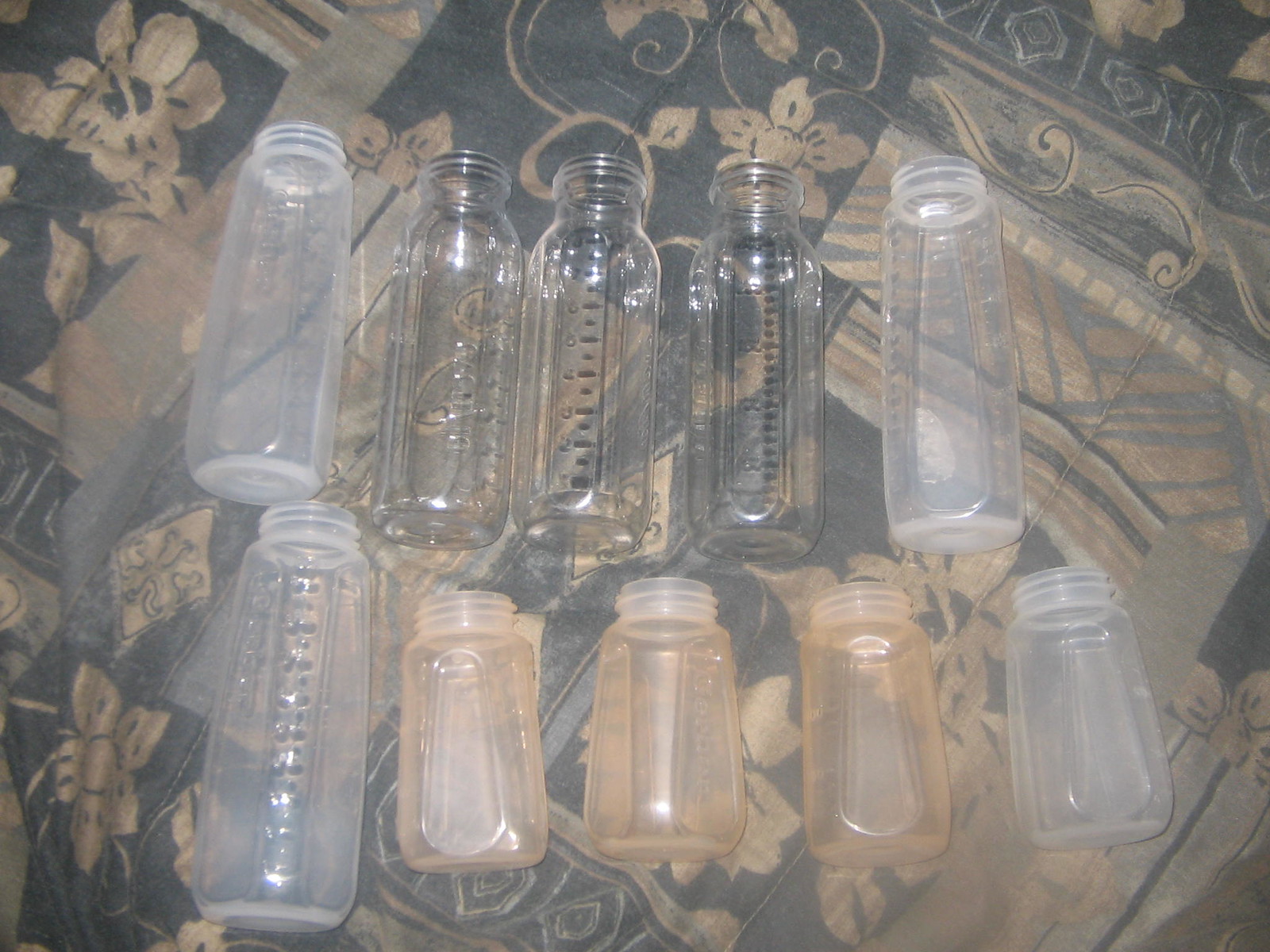This detailed color photograph, taken indoors, features ten baby bottles without their caps or nipples. The bottles are arranged in two rows of five, resting on their sides. The top row consists of five longer bottles, each marked with measurement labels, though the text is not legible. From left to right, the bottles in this row include a translucent one, followed by three clear bottles, and ending with another translucent one. The bottom row also has five bottles: the first one matches the top row in size and translucence, while the remaining four are shorter with no labels. Notably, the next three bottles are made of a brownish clear, or peach-colored plastic, and the final bottle is a translucent white-clear color. All the bottles have a combination of straight and rounded sides, giving them a hexagonal or octagonal shape. This arrangement lies on a quilt with alternating blue and white squares adorned with simple, faded floral designs. The overall color scheme of the photograph appears washed out, adding a muted tone to the scene.